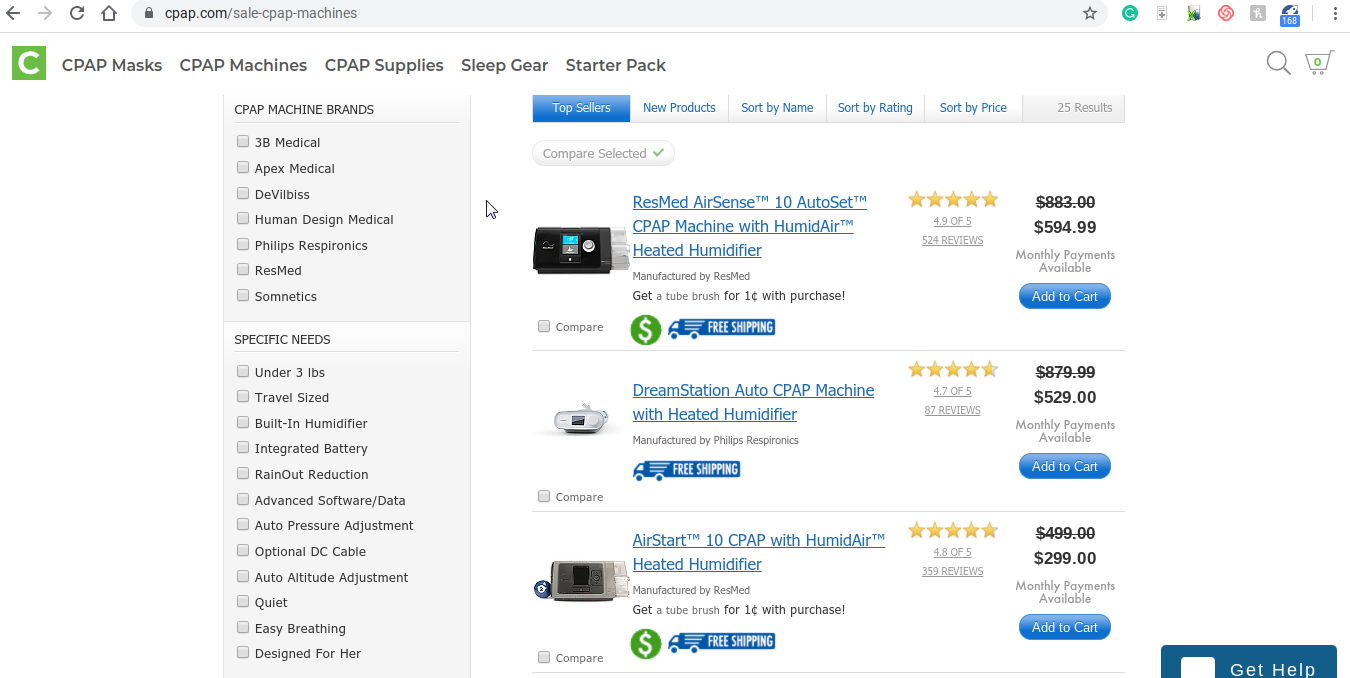The image is a screenshot set against a solid white background, displaying the webpage of CPAP.com’s sale on CPAP machines. In the upper left corner, there's an address bar with the URL "cpap.com/sale-cpap-machines." Below the address bar is a green square with a white "C."

The webpage is organized into various sections: CPAP Masks, CPAP Machines, CPAP Supplies, Sleep Gear, and Starting Pack, distributed across tabs below the main navigation. A prominent blue box with white text highlights "Top Sellers." Other tabs include "New Products," "Sort by Name," "Sort by Rating," and "Sort by Price," with a total of 25 results displayed.

The first product listed is the ResMed AirSense 10 AutoSet CPAP Machine with a HumidAir Heated Humidifier. It has a notable rating of 4.9 out of 5, based on 524 reviews, represented by five yellow stars. The original price of $883 is struck through, indicating a discount. The new price is $594.99 with an option for monthly payments. Below the price, a green circle with a white dollar sign indicates savings, while to its right, an icon of a truck signifies "Free Shipping" in white text against a blue truck image.